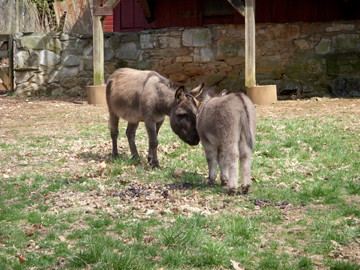The image captures a picturesque, rustic setting featuring two young donkeys in an enclosure. The donkeys, one grayish and the other light brown, stand in the center of a grassy field interspersed with patches of dry, light-colored dirt. Positioned at a 30-degree angle, one donkey faces the camera while the other has its back to it, both appearing to nudge or touch necks. Their tranquility is highlighted against the backdrop of a gray and brown stone wall with a door on the far left. Two wooden pillars, serving as support beams for an unseen veranda, rise vertically in front of this wall, contributing to the overall rustic charm. The scene is further enriched by the subtle details of crisscross lumber emerging from the top of the pillars, hinting at the structure above. Together, the donkeys and their surroundings create a tranquil, bucolic image.